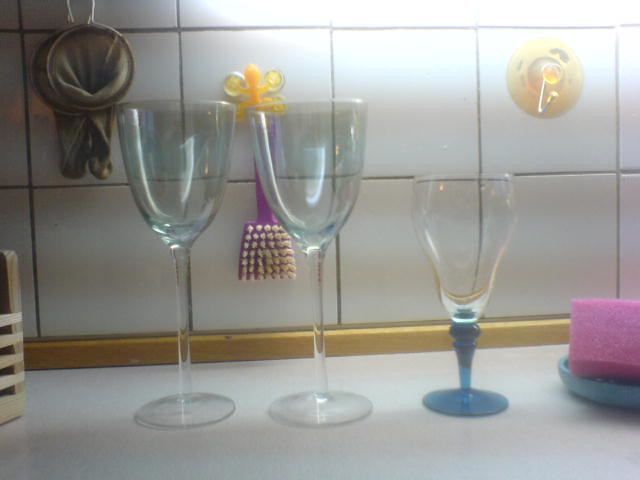The photograph was taken indoors, set on a white countertop with a backdrop of white square tiles. Dominating the scene are three glasses neatly aligned on the counter. The two taller glasses are clear wine glasses, while the third, smaller, glass has a blue base. In the upper left corner, there's a partly visible tea strainer. Adjacent to the glasses on the right, a light blue dish holds a purple sponge. The tiled wall features multiple suction cups, one with a purple brush attached. Additionally, there are some small yellow and bee-shaped items hanging on the wall, adding a touch of character to the otherwise pristine kitchen setting.